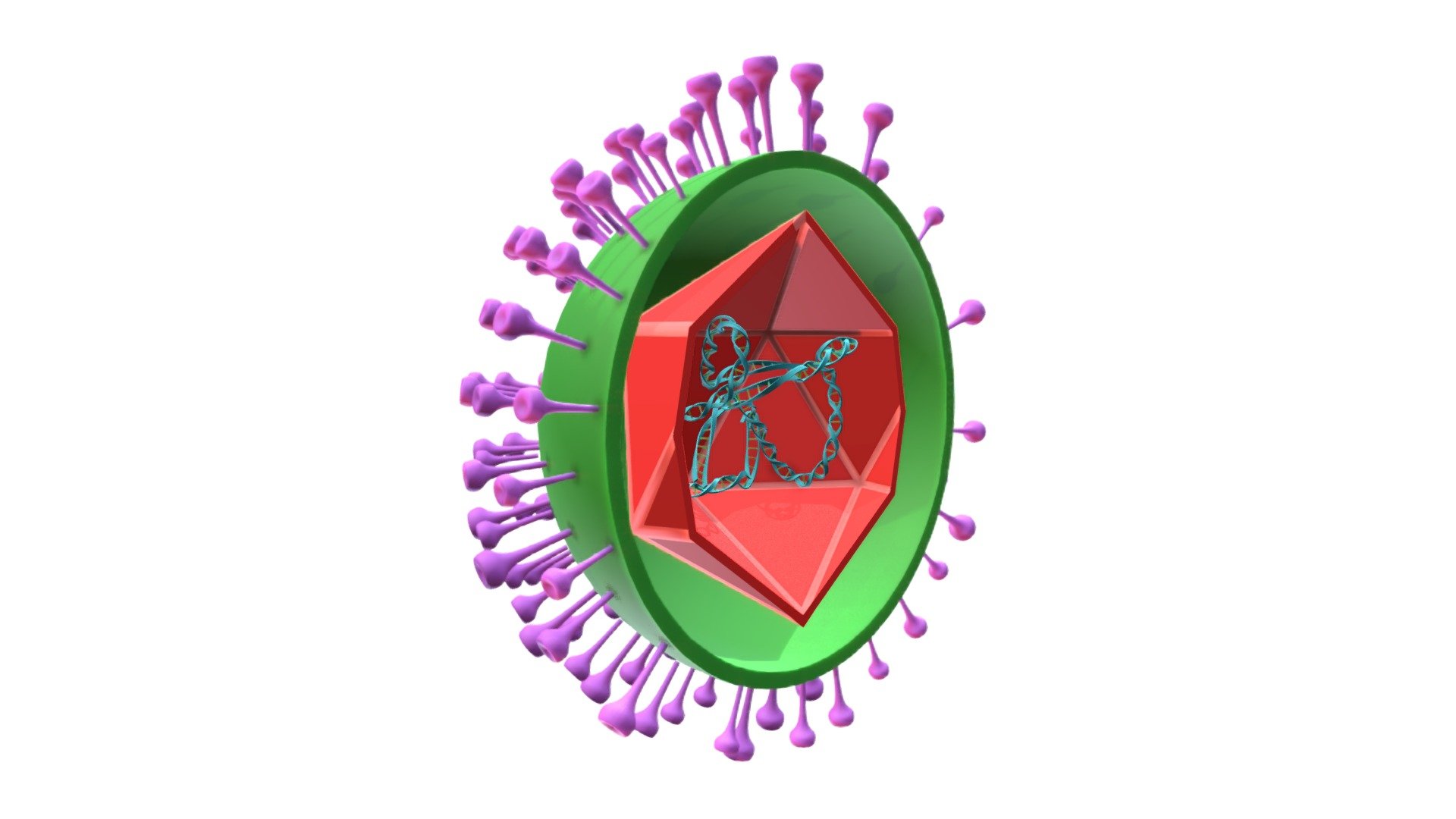The image depicts a detailed, color-illustrated cross-section of a green, spherical object, resembling a cell. The exterior of the green sphere is studded with numerous pinkish-purple protrusions, akin to pushpins or golf ball tees, with widened tips. These spindles, which surround the entire circumference of the sphere, vary in density, with an estimate of at least 50 on the broader sections and around 15 on the thinner areas. Inside the green sphere lies a red, hexagon-like structure, which houses a light blue, twisted, and contorted chain-like object resembling a double helix. The intricate interior elements are vividly displayed, showcasing an anatomy-style diagram cut in half to reveal the inner components.